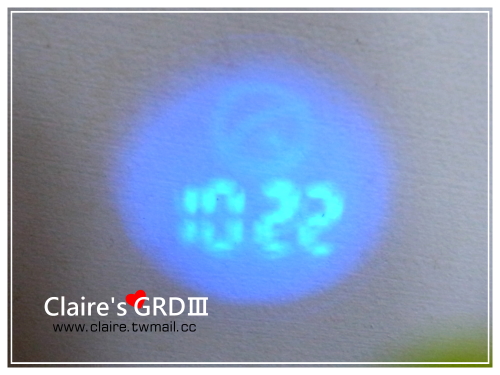This image features an out-of-focus photograph with a graphic in the bottom left corner. The graphic includes the text "Claire's GRD" in capital letters, followed by "III" in Roman numerals. Below this, there is a website URL repeated twice: "www.claire.twmail.cc."

The photograph depicts a lit blue dot, which appears to be backlit and possibly covered with a piece of paper. Above the blue dot is an out-of-focus circular shape that resembles the Death Star from Star Wars, characterized by an orb-like structure with a central horizontal line and a distinct spot on the bottom. Additionally, the number "1022" is visible in the image, which could suggest a time.

For more details or context about the image, visiting the specified website might provide further information.